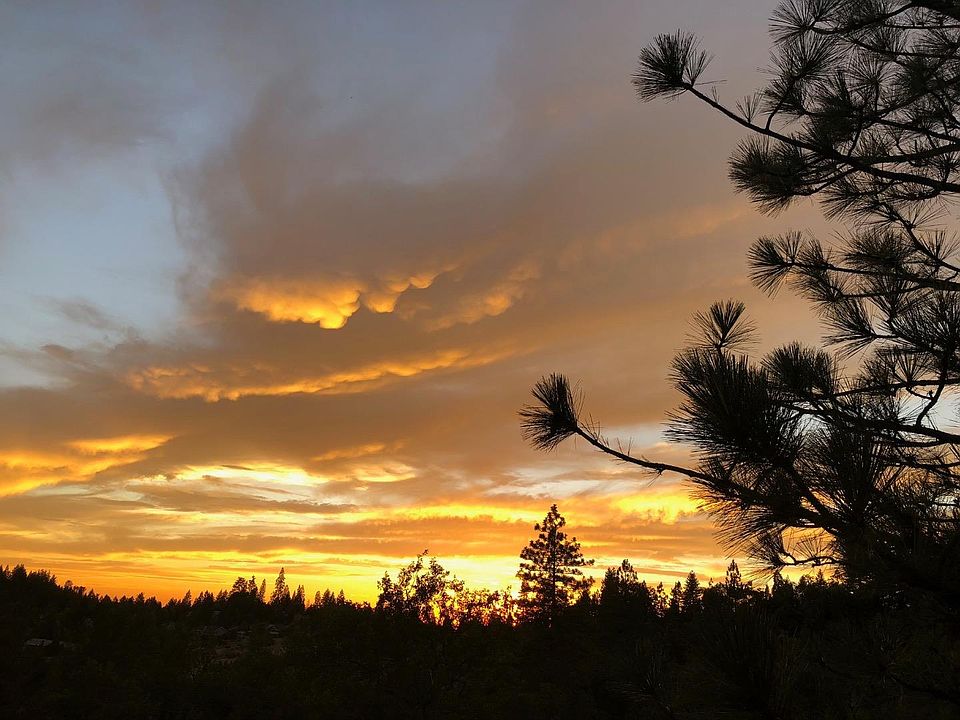A breathtaking photograph captures the serene beauty of a sunset, or possibly a sunrise, over a lush forest. On the right-hand side of the image, the nearest element to the viewer is a towering pine tree with its needle-laden branches silhouetted against the radiant backdrop, appearing almost black due to the light source coming from the front. The entire lower portion of the image features the forest, also rendered in black silhouette, with treetops forming a narrow strip about an inch wide along the bottom, creating a striking contrast to the vibrant sky above.

The sky, dominating the upper three-fourths of the image, unfolds in a mesmerizing gradient of colors. Just above the horizon line, a bright band of yellow and gold bathes the scene in warm, glowing light. Interspersed within this golden expanse are clouds, tinged in shades of burnt orange, seeming to float across the composition. Higher up, the clouds darken into deeper hues of burnt orange and brown but still reveal streaks of bright golden yellow where the sun's light pierces through.

Ascending further, the clouds begin to thin out, transitioning to a more muted gray. In the upper left-hand corner, a faint hint of muted blue sky peeks through, adding a subtle cool tone to the otherwise warm palette. The interplay of light and color in this photograph beautifully encapsulates the tranquil yet dynamic nature of a sunset or sunrise over a forested landscape.